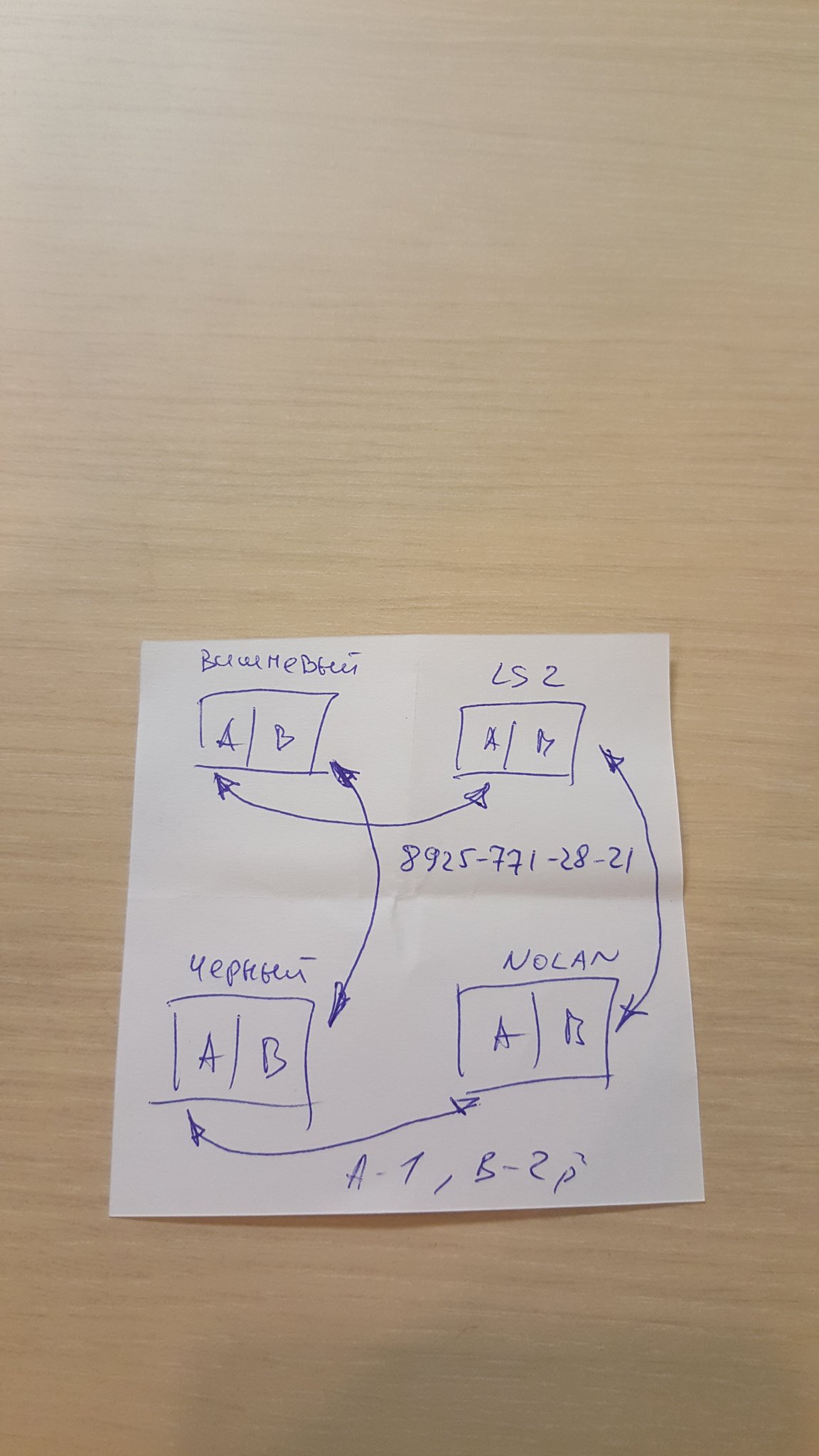The close-up image features a small white square piece of paper positioned slightly off-center on a light wooden tabletop that extends from the top to the bottom of the frame. The paper appears to have been written on with a blue pen and contains various labeled sections and graphical elements. 

In the lower center of the paper, there are two squares side by side, each labeled "A" and "B." There is a central title at the top of these squares, although it is somewhat difficult to decipher due to the cursive script. 

To the right of these squares is another pair of squares, also labeled "A" and "B," with "LS2" written as a top title. These squares are connected to the ones below them with arrows, and they have an overarching title of "Nolan" at the top.

Towards the right center of the paper, there is a numerical sequence: "8925-771-28-21." At the bottom center, there is an alphanumeric notation: "A-1," followed by "B-2P." This written structure suggests some sort of informational or diagrammatic representation.